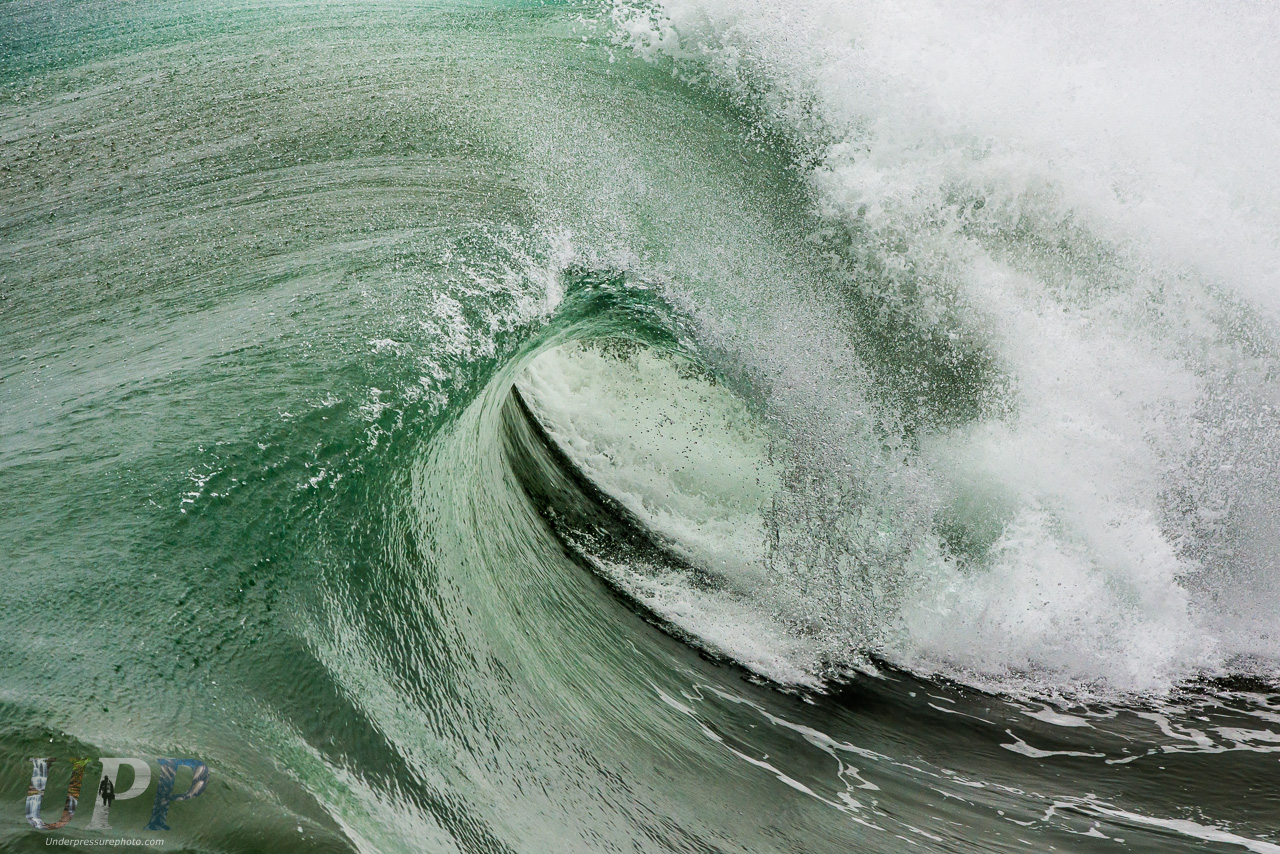The photograph captures a stunning, large wave in vibrant green-blue hues, perfect for surfers seeking the ultimate barrel shot. The wave, with darker shades where the water deepens and lighter, clearer tones where sunlight hits, curls dramatically as it crashes. On the left, the ocean forms the wave that beautifully crests and mists with white frothy water at the top right. In the lower left corner, the logo "UPP" or "underpressurephoto.com" is visible, featuring distinct patterns, possibly including an American flag and military figures, though the exact meaning of the logo remains unclear. The image is taken during the day, with daylight reflecting off the dynamic, curling tidal wave.